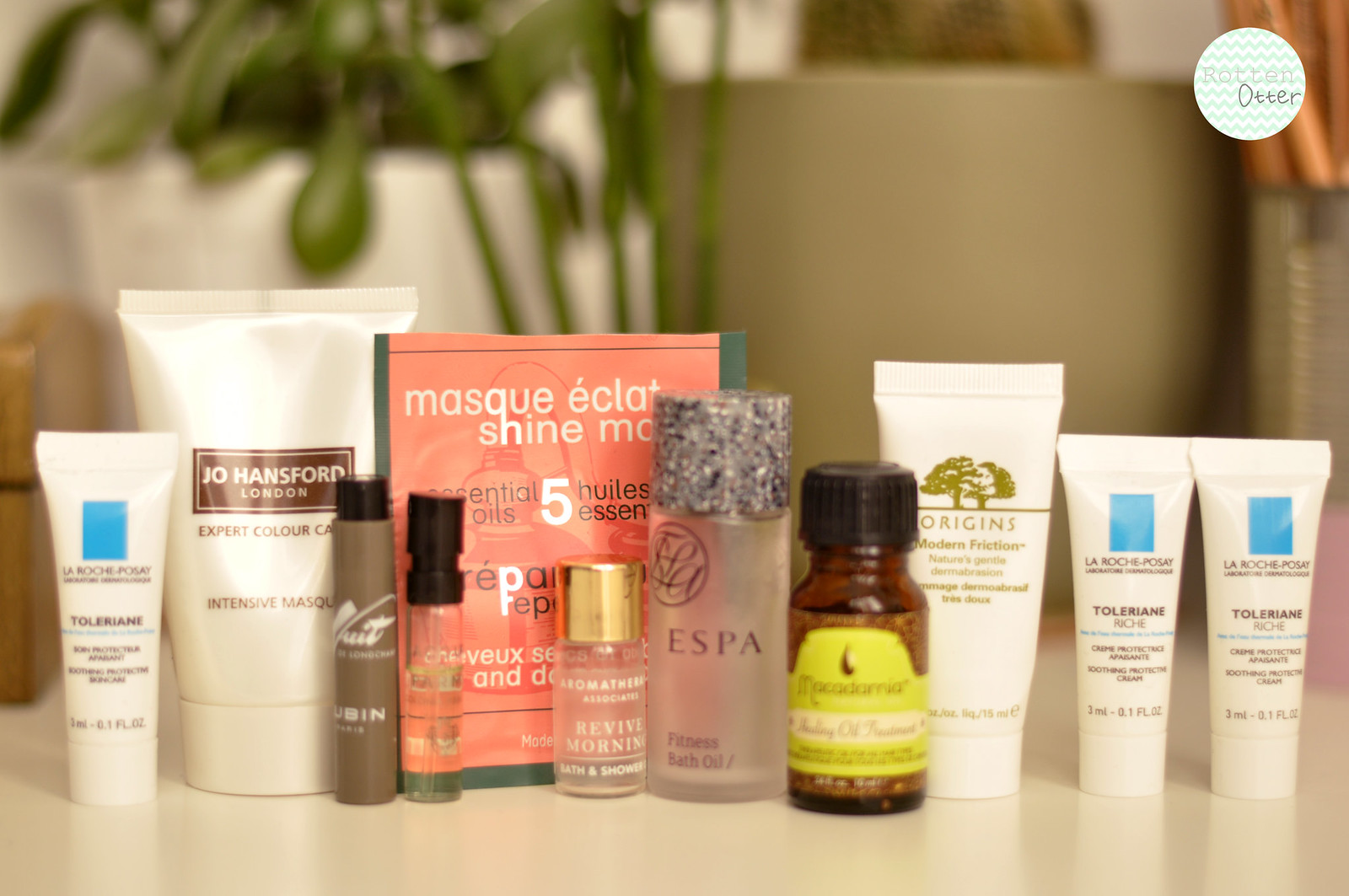A bright photograph showcases an array of sample-sized skincare products arranged neatly on a pristine white counter. In the background, a subtle blur reveals hints of gray and white potted plants, adding an organic touch to the setting. Dominating the top right corner, a circular logo features prominently, displaying the brand name "Rotten Otter" in light blue chevron on a white background.

The assortment includes well-known names like Origins and ESPA. The ESPA product stands out in a small glass bottle with a distinctive green topper. Nearby, a vibrant pink package labeled "Mask Shine" suggests a luxurious face mask, adding a pop of color to the otherwise muted palette.

Additional products include a small sample from Johansford, London, and another item where the partial text reads "LA," leaving a hint of mystery. Some bottles are crafted from glass, boasting a sleek, delicate appearance, while others come in slightly taller, white squeeze containers, emphasizing practicality and ease of use. Each item in this mini collection represents a different aspect of facial care, from lotions to cleansers, encapsulated in chic, travel-friendly packaging.